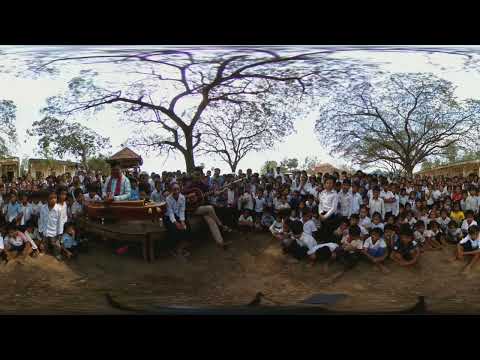The image is a completely black square, with no discernible features, text, objects, or colors present. It looks like a still frame from a show, a YouTube video, or perhaps even a simple wallpaper. The image measures roughly three to four inches in height and width, giving it the appearance of a perfect or near-perfect square. On a computer screen, especially against a white background, it creates the illusion of a deep void or black hole, as if something might leap out or you could fall into it. This dark and hollow appearance can seem endless until you touch the screen and realize it's just an image. The simplicity and uniformity make it an easily describable yet striking visual experience, akin to staring into nothingness.